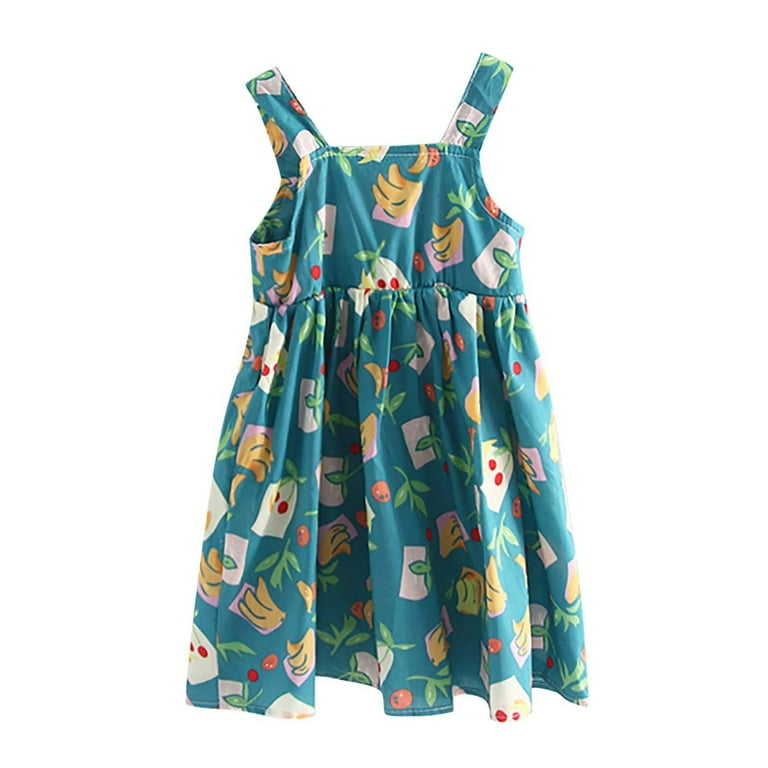This image depicts a little turquoise dress, likely for a young girl, displayed against a white background. The sleeveless dress features thick straps and is designed with an elastic cinch just below the chest area, giving it a slightly flared silhouette. The dress is adorned with vibrant and whimsical fruit patterns, including bananas, cherries, green leaves, and some cartoony elements like purple squares and red dots. Scattered across the light blue fabric are additional images resembling white and beige envelopes with fruit motifs atop them. The dress's colorful and busy design makes it a cheerful and playful garment that would likely come down to the knee of a young child.